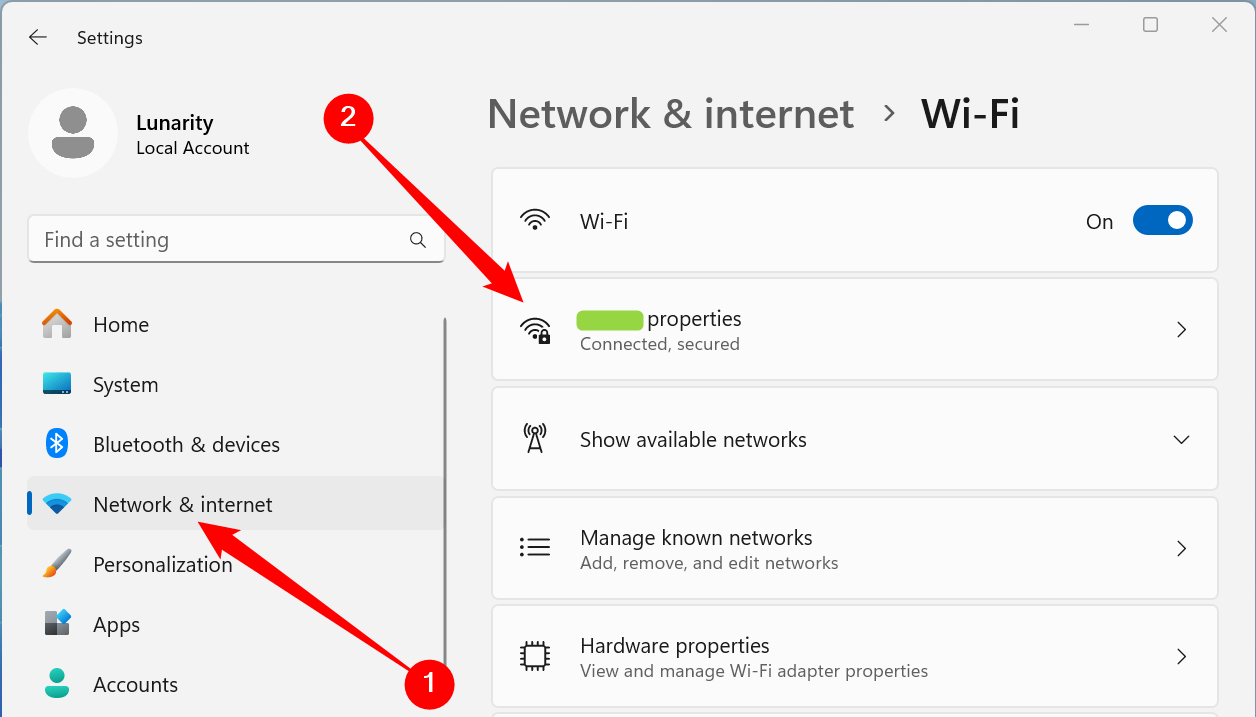A detailed settings page for a Wi-Fi device is depicted. At the top-left corner, a gray arrow is pointing left and beside it, the word “Settings” is prominently displayed. Below this, the user profile is shown with the label “Lunarity Local Account” next to a profile icon. 

Underneath the profile information is a search bar labeled “Find a setting.” Following this search bar is a navigation menu displaying multiple options, each accompanied by corresponding icons: 
- Home (house icon)
- System
- Bluetooth and devices
- Network and internet (highlighted with a red circle containing the number one)
- Personalization
- Apps
- Accounts

The highlighted "Network and Internet" section has a red circle with the number one next to it, indicating it is currently selected. Additionally, across the top part of this section, a red circle with the number two and an arrow pointing to the right is visible, which indicates focus on a specific feature.

On the right-hand side of the screen, details under the headline "Network and Internet" are shown:
- The word “Wi-Fi” is displayed at the top-left, next to a blue toggle switch that is in the "On" position.
- Below "Wi-Fi" is the word “Properties” next to a green line, below which it says “Connected and secured.”
- Additional options listed are “Show available networks,” “Manage known networks,” and “Hardware properties,” each with brief descriptive text.

The layout is clear and organized, ensuring that users can easily access and manage their Wi-Fi settings.